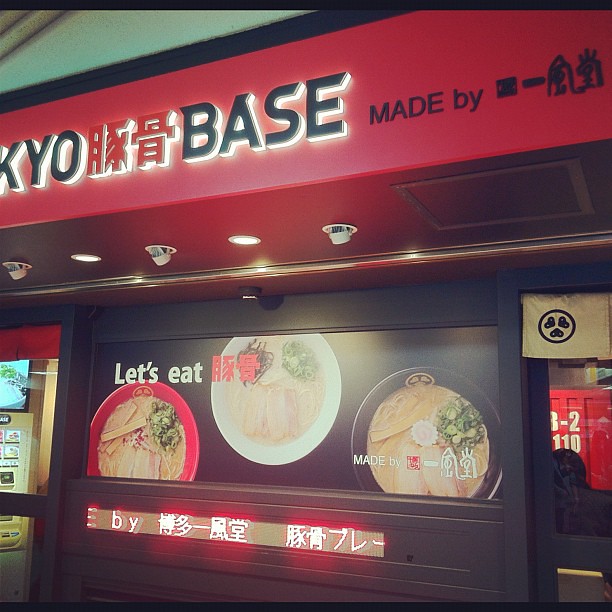The photograph depicts the exterior of an Asian restaurant, likely Japanese or Korean, featuring a striking red metal sign at the top displaying "KYO Base" in illuminated black neon letters. Red neon characters, possibly Korean or Japanese, are situated between the words "KYO" and "Base." To the right of this sign, in black neon, it reads "Made By" with additional Asian characters. Below, a dark black wall showcases a digital display banner saying "Let's Eat," flanked by images of various dishes in red, white, and black bowls. Above the bowls, Japanese characters in red are also visible. The awning is adorned with ceiling lights that illuminate the sign and the large screen displaying the menu or promotional phrases. The storefront includes a black door with windows on either side, set against a white ceiling, and a light green triangular section above it.